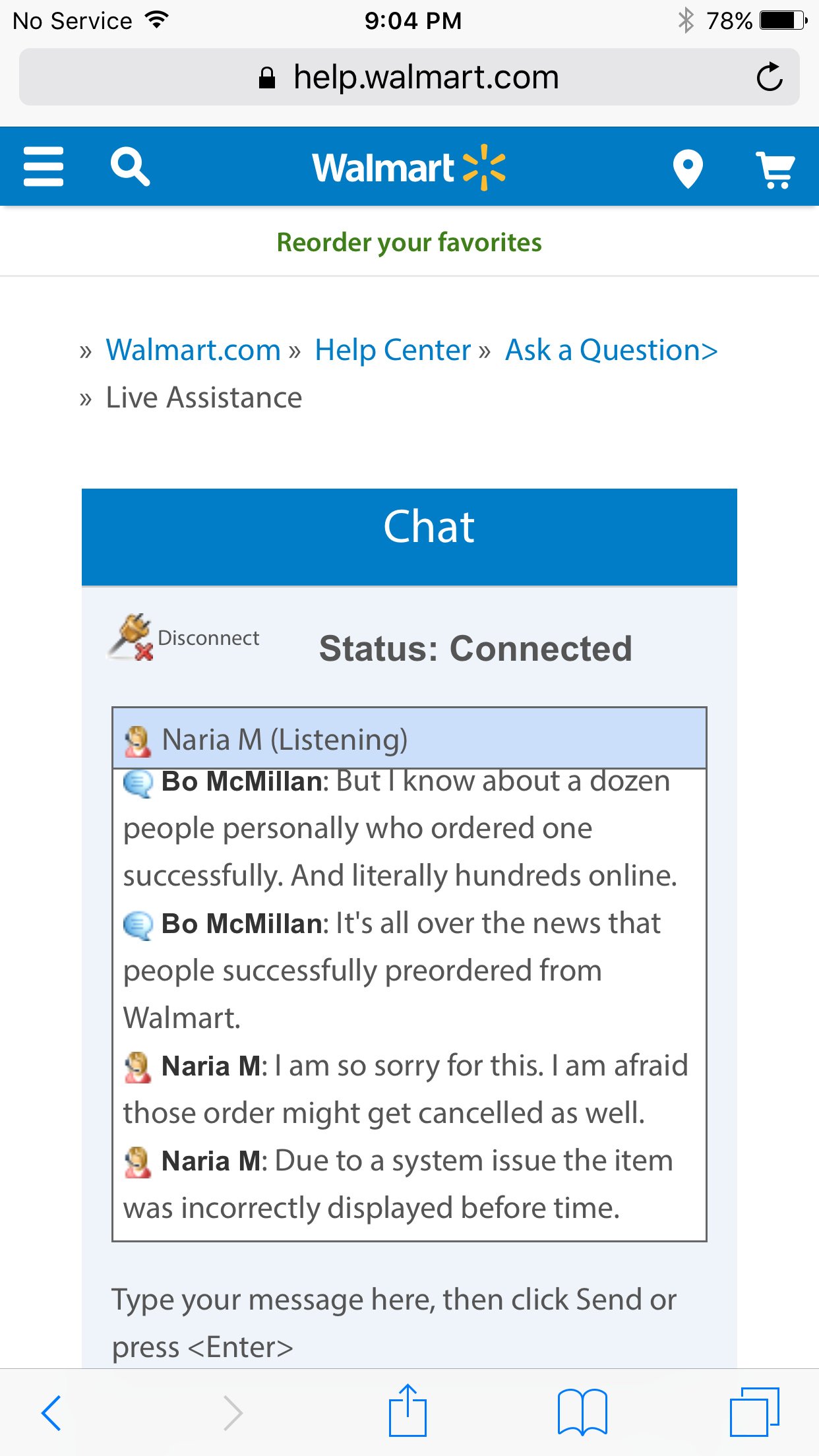A detailed image description of a Walmart.com help page displayed on a user's smartphone:

The image shows a Walmart.com help page on a user's cell phone screen. The top left corner of the image displays the text "No Service" in black, indicating a lack of cellular signal, while the top right corner shows the time as "9:04 PM" and a battery life indicator at 78% on a light blue background.

Beneath this, a darker banner contains the URL "help.walmart.com" with a refresh arrow and a padlock icon placed to the left of the URL, indicating a secure connection.

Next, there is a bright blue horizontal banner with the Walmart logo, an orange starburst, and the text "Walmart" in the center. On this same banner, a magnifying glass icon for search is situated to the left, followed by a three-bar menu icon. To the right of the Walmart logo, there is a location icon, and further right, a shopping cart icon.

Underneath the blue banner, the text "Reorder Your Favorites" appears in black on a white background. Below this, on the same white background, "Walmart.com" is displayed in bright blue, followed by an arrow pointing to the right with the text "Help Center" in bright blue. Adjacent to this is the phrase "Ask a Question" also in bright blue. Below these options, "Live Assistance" is written in gray.

Following this, there is a smaller rectangular chat box. At the top of this chat box, a bright blue banner displays the word "Chat" in white. Directly below this, on a light blue background, the status is indicated as "Status: Connected" in black text, with an option to "Disconnect" in tiny letters next to it.

The chat box contains ongoing conversation. A representative named Naria M, indicated as "Listening" in parentheses, is engaging with the customer. The customer, Bo McMillan, has his name in bold black text. His messages include expressions of frustration, stating, "But I know about a dozen people personally who ordered one successfully and literally hundreds online," and, "It's all over the news that people successfully preordered from Walmart." Naria M has responded with two apologies.